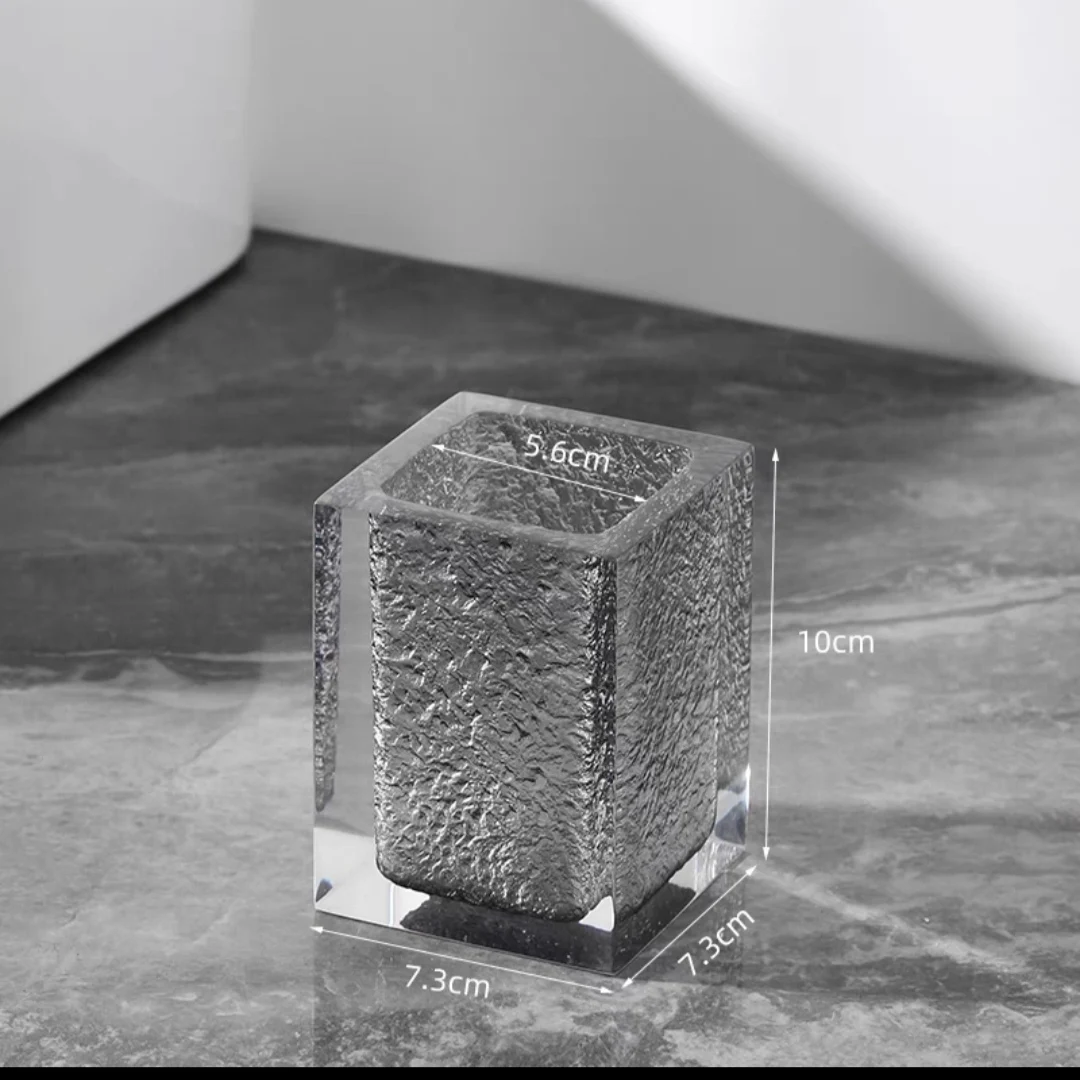The image features a glass cube with smooth exteriors, resting on a dark gray and light gray marble table. The glass cube displays various measurements: the diameter is 5.6 centimeters, the standing height is 10 centimeters, and the base measures 7.3 centimeters. Inside the cube, a silver or dark gray metallic object can be seen, which appears uneven and fluffy, somewhat resembling crumpled aluminum foil. The background consists of partial white walls, casting shadows onto each other and the marble table below. The photograph is monochromatic, lacking any colors besides shades of black, white, and gray.